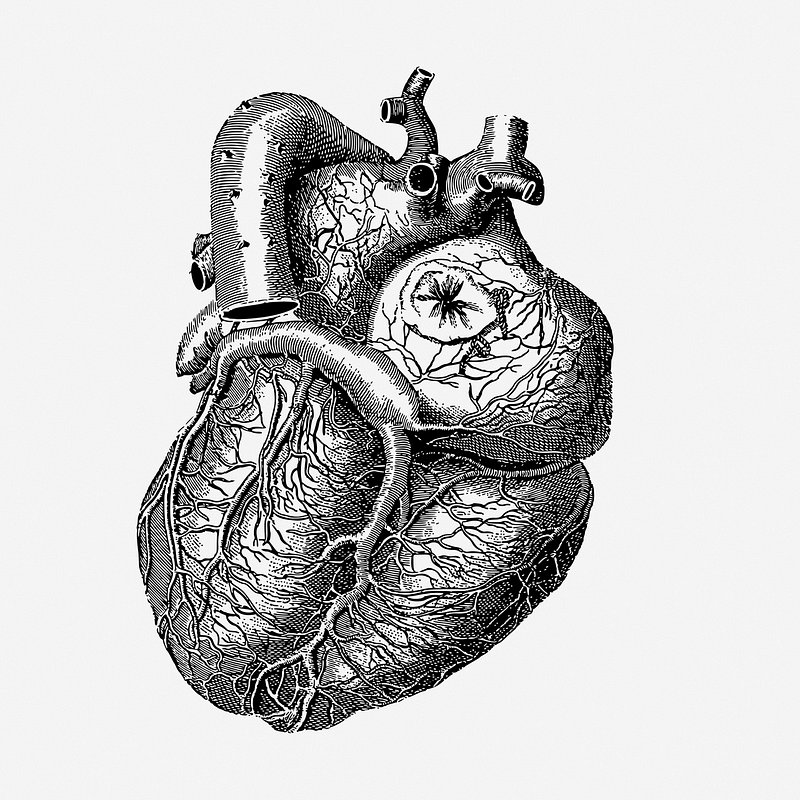This is a highly detailed, black-and-white anatomical illustration of a human heart, drawn with meticulous line work on a white background. The heart, rendered in black ink, showcases an intricate network of veins and arteries. Various tubes and valves protrude from the top, with a notably large pipe-like structure extending downwards. The illustration gives the impression of being crafted digitally due to its slight pixelation. The heart is surrounded by numerous veins, creating the appearance of a complex circulatory system enveloping it. The middle of the heart features a prominent vein, adding to the detailed depiction of its internal structures.